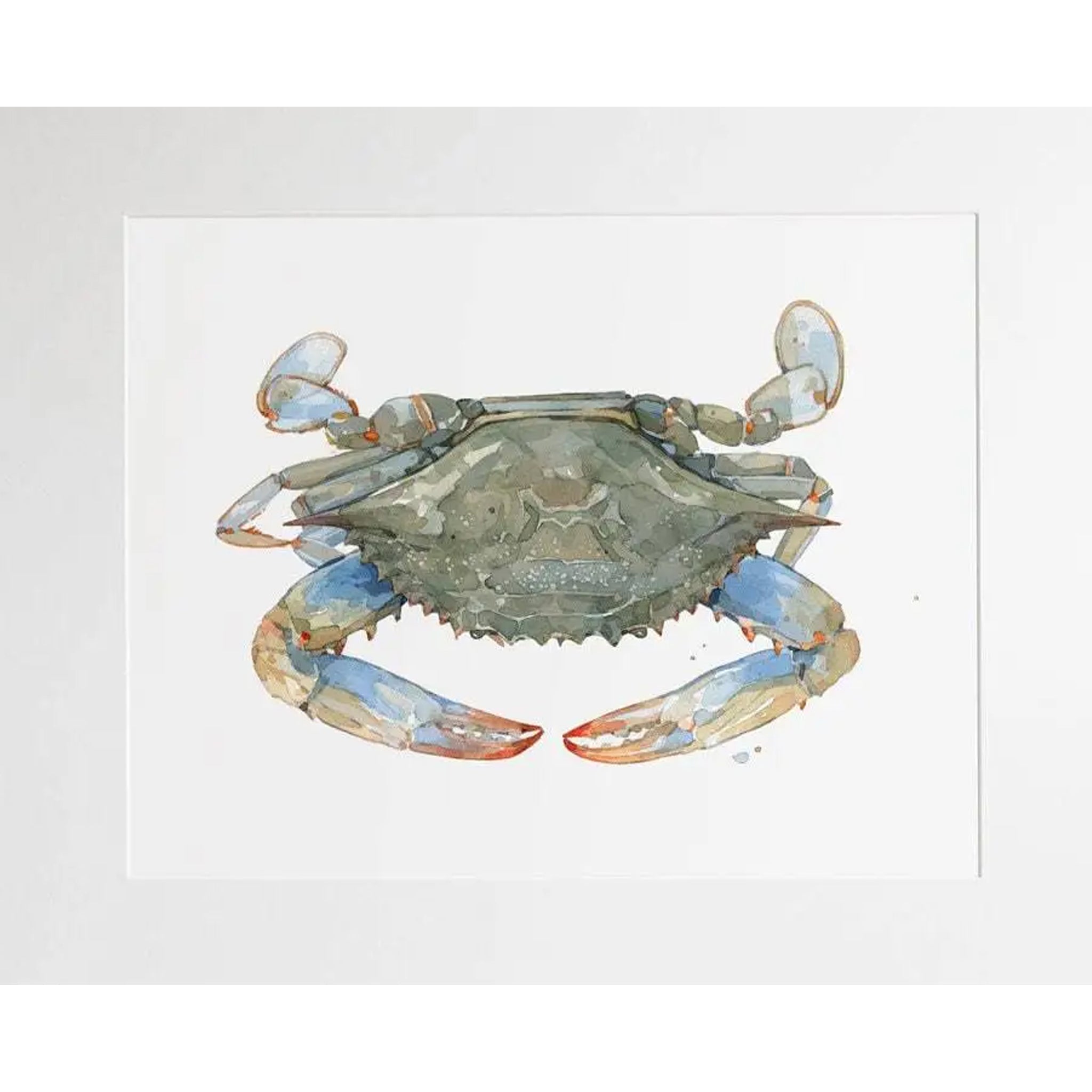This image showcases a detailed, watercolor painting of a crab, framed within a simple white rectangular frame. The crab is centered on a white piece of paper, which is bordered by a light gray frame approximately three-quarters of an inch thick. The crab features a light green shell with nuances of gray, blue, yellow, and red. The crab's legs and pinchers exhibit a mix of colors: the front pinchers are predominantly red, while the legs towards the back are tinted with blue, gray, and hints of brown. There are four pinchers with distinct blue and red highlights. Scattered across the white background near the right side of the crab are five gray splotches, possibly paint drips, adding an organic touch to the artwork. The illustration captures a vivid and somewhat abstract representation of the crab, emphasizing its unique coloration and the artistic medium.